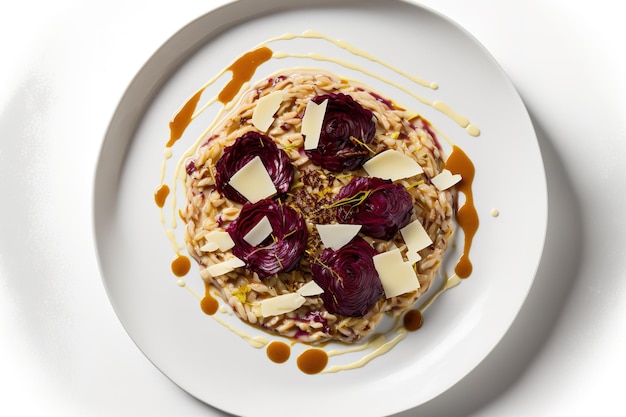This photo, taken from a top-down perspective, showcases an intricately plated dish on a circular white plate set against a cream-colored background with subtle shadows. The centerpiece of the dish is a tight circle of grains, varying from light to dark brown in color. Adorning this are five drops of a purplish-maroon paste, likely beet or red cabbage hearts, arranged artistically around the grains. Interspersed are very thin slices of creamy-colored cheese and a few sprigs of herbs. A distinctive element is the drizzle of syrup, both dark brown and light cream-colored, encircling the dish. The overall presentation is elegant, turning a simple grain-based dish into a gourmet experience.